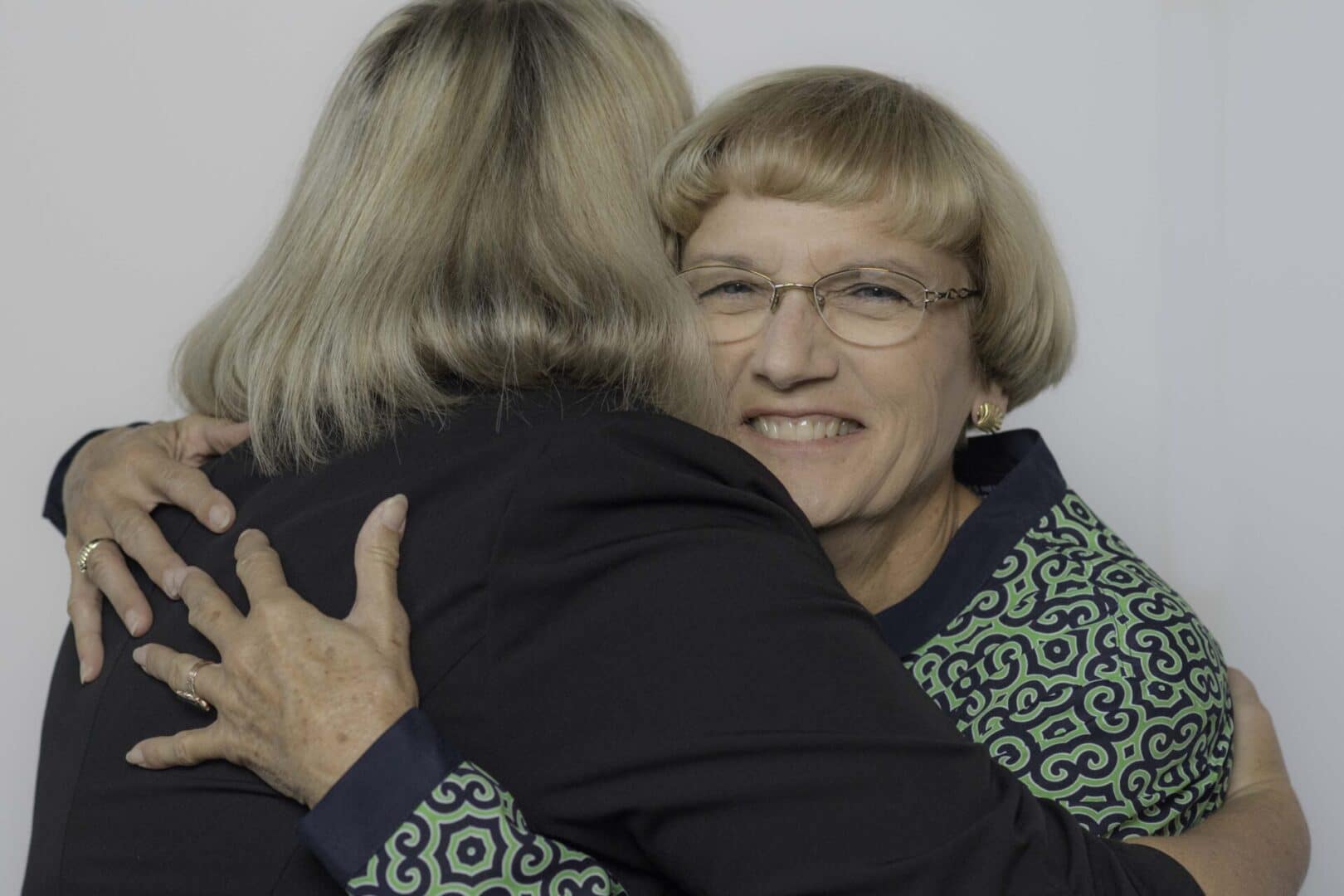A touching moment captured in an image of two people embracing against a flat, gray-colored wall. The person on the left, who has their back to the camera, is wearing a long-sleeved black jacket and has blond hair with dark streaks. They have their arm around a woman who appears to be around 60 years old. She is beaming with a wide smile, showing her teeth, and is wearing thinly-rimmed glasses. Her short bob haircut is blond, and she is adorned with gold earrings. Her outfit features a green and blue patterned shirt with a navy-blue collar and wrist cuffs. Additionally, she is wearing a gold ring on one of her fingers, completing her look.